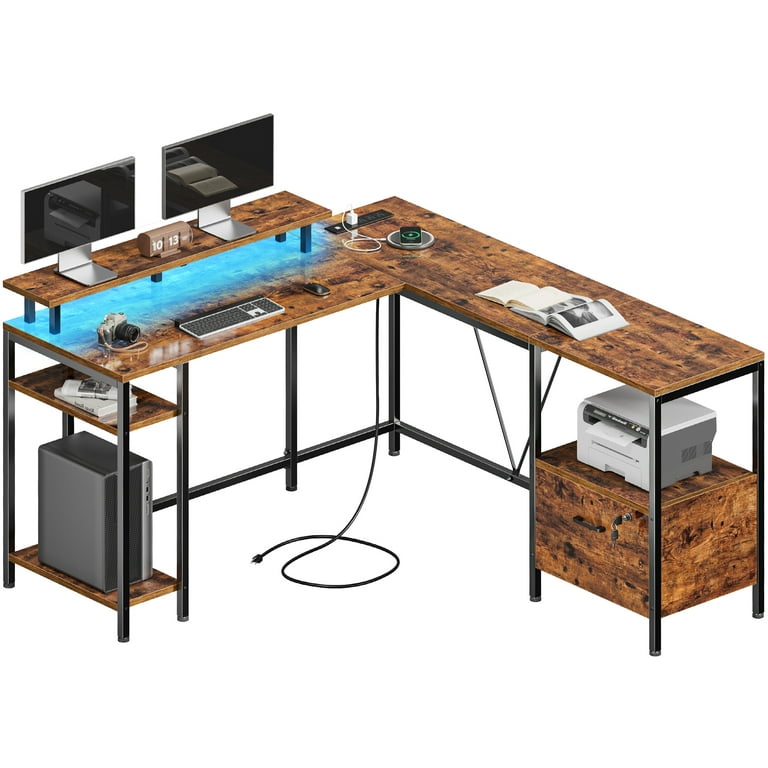The image depicts a detailed, computer-generated workstation setup featuring an L-shaped desk designed to fit perfectly in a corner. The desk has an upper tier supporting two computer monitors with black screens and reflections, flanked by blue LED under-lighting. Positioned between the monitors is a clock. The lower tier of the desk holds a keyboard, mouse, and a camera seated on a stand to the left of the keyboard. 

Further to the right is an additional attached desk section bearing two open books and a power strip leading to a mat where a phone appears to be charging wirelessly. The desk includes a smaller shelf below, designed to house a desktop computer, as well as a space on the right side with a printer and adjacent storage drawers. Various cords and cables are visible, trailing from beneath the desk. The entire workstation is framed with a black metal structure, set against a white background, with the desk itself boasting a wooden finish.